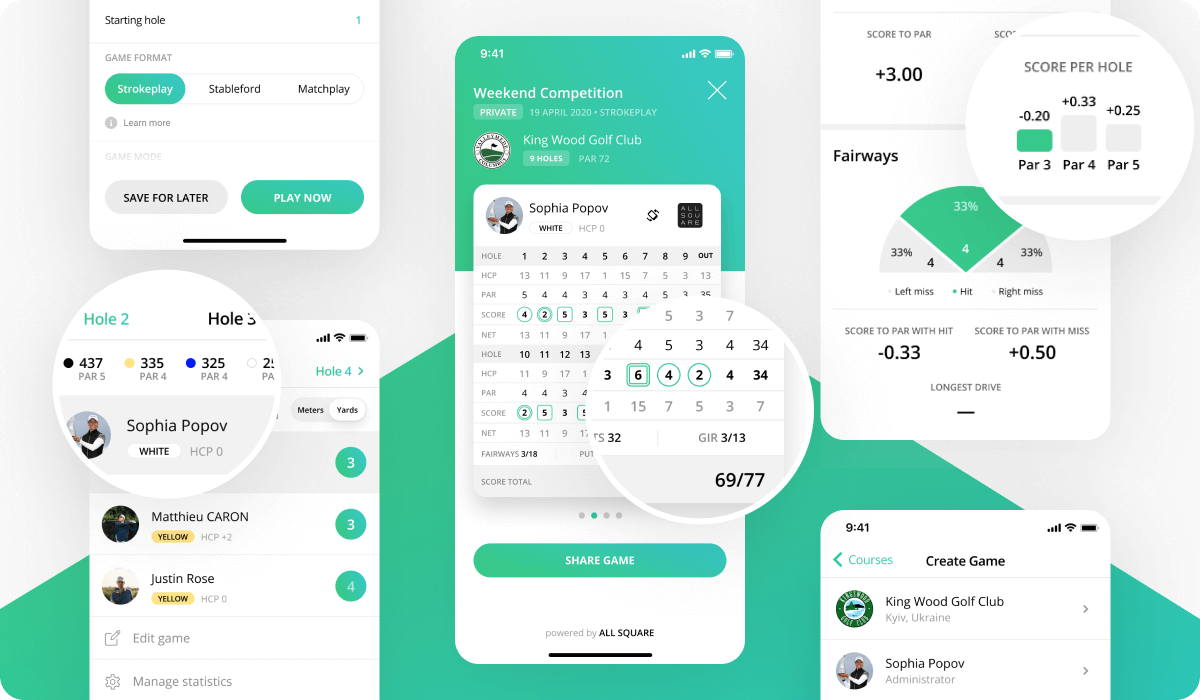In this captivating image, five cell phone screens are prominently displayed, all facing the viewer. Each screen showcases a specialized golf application designed to track users' golf scores and record the history of their previous games. Key layout elements such as "par 3," "par 4," and "par 5" are visible, indicating the complexity and variety of the courses. Notable details include a specific mention of hole number 3 on one of the screens and highlighted circular sections that provide a magnified view of certain application features.

One screen prominently features a "weekend competition" option, while another screen displays the functionality to "create a game." Additionally, users can select to view specific holes on the golf course through the app. The arrangement of the phones is well-organized: one screen occupies the center position, flanked by two screens on each side, creating a symmetrical and engaging presentation.